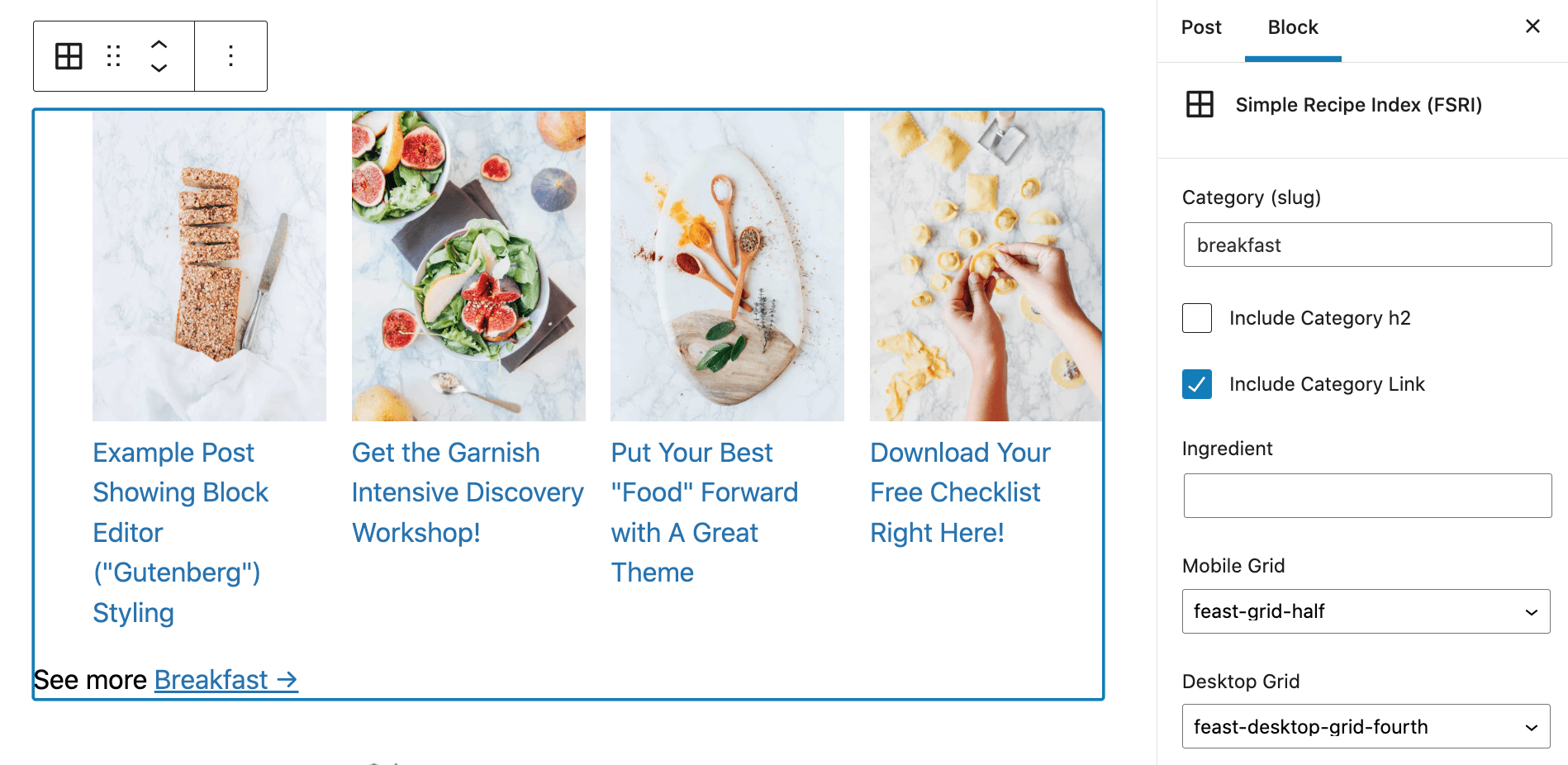Upon first glance, the page appears to be either a cooking or editing platform. Dominating the left side is a large square outlined in blue, containing four distinct images.

1. The top image depicts a sliced loaf of bread aligned vertically with a knife positioned to its right. A caption beneath reads, "Example post showing block editor, Gutenberg styling," indicating an instructional post on item posting. The text is hyperlinked in blue.
   
2. Below it, an image features two vibrant salads on a marble surface, accompanied by various garnishes including a red fruit laden with seeds and a silver spoon. The adjacent caption promotes a "Garnish Intensive Discovery Workshop," also a clickable link.

3. The following image presents a wooden cutting board with four wooden spoons, each containing different spices. The caption urges, "Put your best 'food' forward, with a great theme," with 'food' in quotation marks. The phrase is hyperlinked.

4. The last image shows hands meticulously crafting various shapes of pierogies, both circular and square. The caption invites users to "Download your free checklist right here," and includes another hyperlink.

Beneath these images is an additional line stating "See more" in black, followed by "Breakfast" in blue, which is also clickable.

On the right-hand side of the page, labeled "Post block," there is a horizontal blue line indicating the current position. Below, a square divided into four sections is labeled:

- "Simple Recipe Index (FRSI)"
- "Category: slug (Breakfast)"
- An unchecked box labeled "Include Category H2"
- A checked box, blue with a white tick, labeled "Include Category Link"

Further down are fields for "Ingredient," which is currently empty, and "Mobile Grid," set to "Feast-Grid-Half" from a drop-down box. Similarly, "Desktop Grid" is set to "Feast-Desktop-Grid-Fourth" from another drop-down box. No additional information is provided.